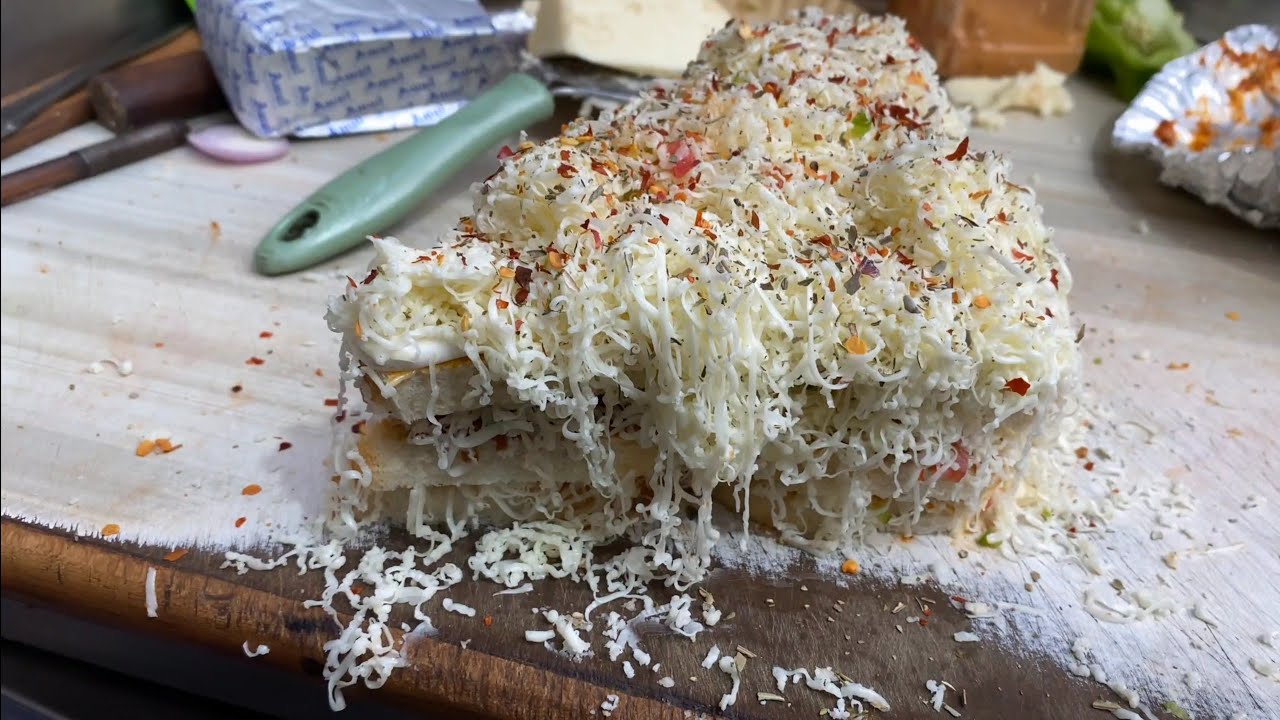This is a detailed color photograph showcasing a cluttered kitchen countertop, with the central focus being a triangular wedge of an indistinct food item, possibly a piece of cake, a layered sandwich, or a slice of lasagna. The food item is heavily obscured by a dense layer of hand-grated white cheese, accompanied by flecks of red and green spices and herbs. The cheese almost overpowers the dish, with pieces of it tumbling onto the well-used wooden surface beneath. In the disorganized backdrop, there are various kitchen items including a cheese grater, a block of cheese, and a piece of tin foil smeared with what appears to be a red, marinara-like sauce. The overall scene suggests recent food preparation, with an emphasis on the abundant use of cheese, appealing to any cheese lover. The image is broader than it is tall, presenting a compressed snapshot of this culinary mess, yet no people are present in the frame.